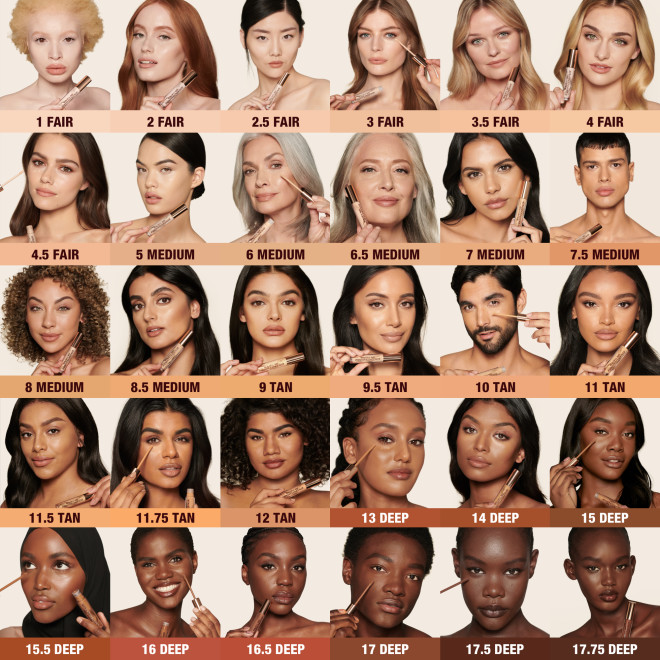This is a detailed composite photograph featuring a grid of approximately 30 models, predominantly female with a couple of males, showcasing a diverse spectrum of skin tones for a makeup brand. The image is organized into rows, each row containing six faces, with each face representing a specific shade of foundation. The shades range from light to dark, starting with "fair" and progressing through "medium," "tan," and finally "deep." The very top row showcases shades labeled from 1 fair to 4 fair. The immediate row below continues from 4.5 fair to 7.5 medium. The third row transitions into darker tones, labeled from 8 medium to 11 tan, followed by the fourth row with labels from 11.5 tan to 15 deep. The final row includes the darkest tones, ranging from 15.5 deep to 17.75 deep. This comprehensive display aims to assist consumers in selecting foundation shades that closely match their skin tones, offering a visual representation that spans from very light complexions to deep ebony hues.